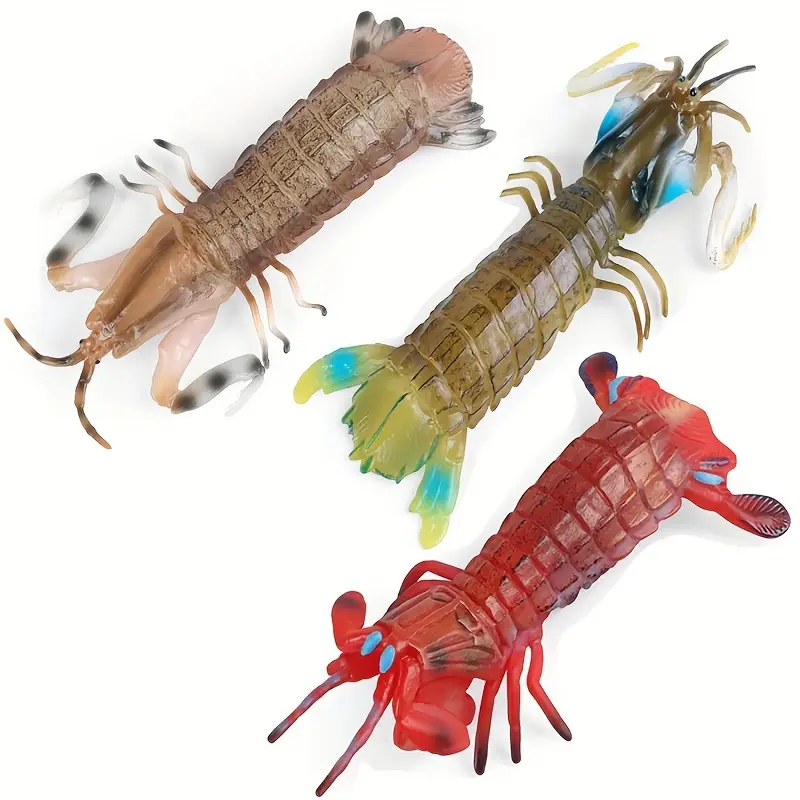This image features three intricately detailed, bug-like creatures arranged in a diagonal row on a pure white backdrop. The creatures, possibly crafted from gummy candy, resin, or even fishing lure material, share common attributes like elongated bodies, multiple legs, and delicate antennae, though each comes in distinct colors and details, hinting at imaginative or fantastical origins.

The top creature resembles a hybrid between a small spider and a moth, featuring an elongated brown body, eight legs, and antennae. Its tan hue is accented with hints of black and white, creating an earthy, natural look.

The middle creature, similar in structure, sports a predominantly green body with blue markings. It also has six legs and antennae, and its appearance is accentuated with a darker yellowish-brown tail and hinting at a light blue, white, and yellowish-brown color on its front legs.

The bottom creature is the most vivid, colored in rich red with noticeable blue eyes and no antennae. It boasts a pair of pinchers at the front of its face, further differentiating it from the others. Blue and possibly cream or dark black shades mix into its coloration, adding to its striking visual appeal. This one faces to the left like the top brown creature, whereas the middle one faces to the right, adding a dynamic orientation to the trio.